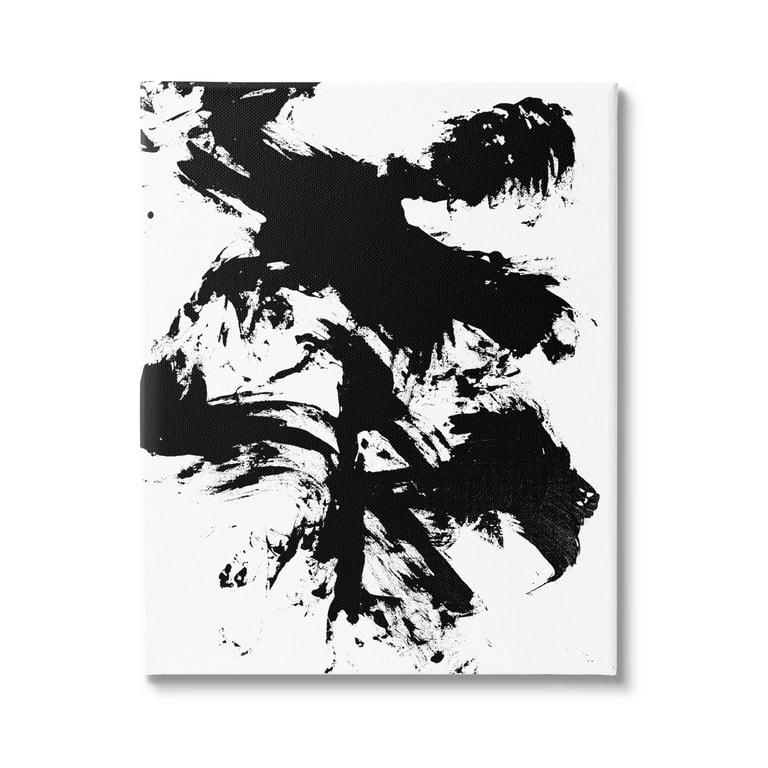This vertically aligned rectangular image depicts a piece of contemporary abstract art on a solid white canvas. The background is solid white, blending seamlessly with the canvas itself, creating an almost ethereal effect. The painting prominently features black paint applied in various methods, including splattering, brushing, and splashing, covering approximately half of the canvas. The top portion showcases a significant black blotch with some splatters that create hair-like shapes. In the center, the black paint forms an impression that could be interpreted as a face, and towards the bottom, the brushstrokes resemble the silhouette of a V-shape and potentially a horse's head. There is no border or text on the canvas, and subtle shadows are visible on the right and bottom edges, adding depth to the image. Overall, the artwork is highly abstract, emphasizing the performative nature of the painter's actions.